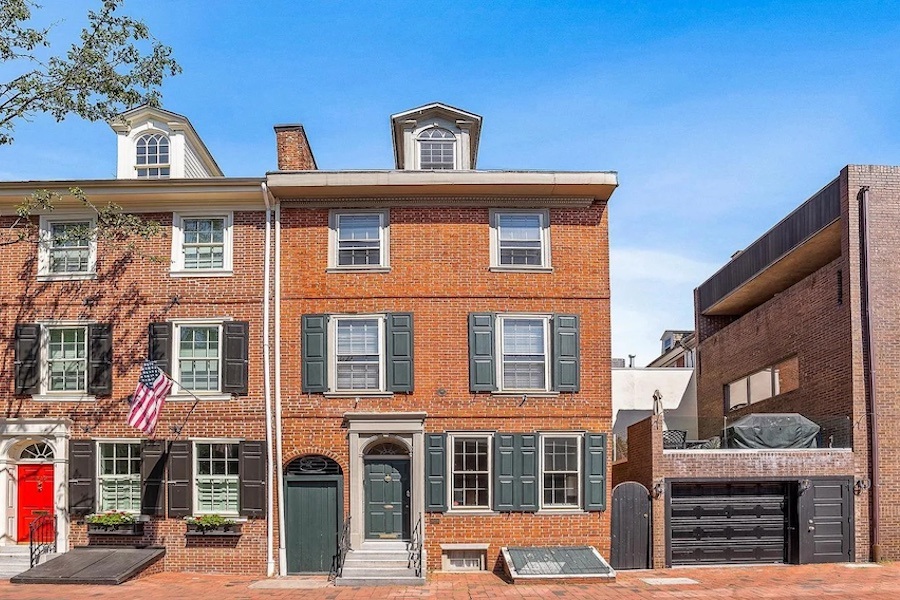This horizontal rectangular image features two adjacent red brick townhouses situated in a city. Both structures are three stories tall and share architectural similarities but exhibit distinct exterior differences. In the foreground, a bright blue sky punctuated by a single wispy white cloud spans the background, while thin branches with sparse flowers or leaves occupy the upper left corner of the frame.

On the left side of the image is the first townhouse, built from lighter red brick. It features a prominent white archway surrounding a bright red door and has an American flag displayed below the second-floor window. Each floor of this townhouse has two windows, framed by light black shutters, and is capped with dormers housing small windows at the roofline. At ground level, an old access chute, reminiscent of historic coal chutes, is visible, suggesting access to a basement area. Abutting this building to the left is a dark brown garage door.

The adjacent townhouse on the right also stands three stories tall, with its slightly darker red brick facade and gray accents. The primary entrance is marked by a gray door within a matching gray archway. This building mirrors the window layout of its neighbor, with two windows per floor, each trimmed in gray shutters. Additionally, a smaller gray door and another gray door on the side are present. Between this townhouse and the garage to its right, there is a small wooden door.

Overall, the scene captures the charming complexity and historical detail of these urban dwellings, highlighting their layered histories through architectural nuances and differing external finishes.